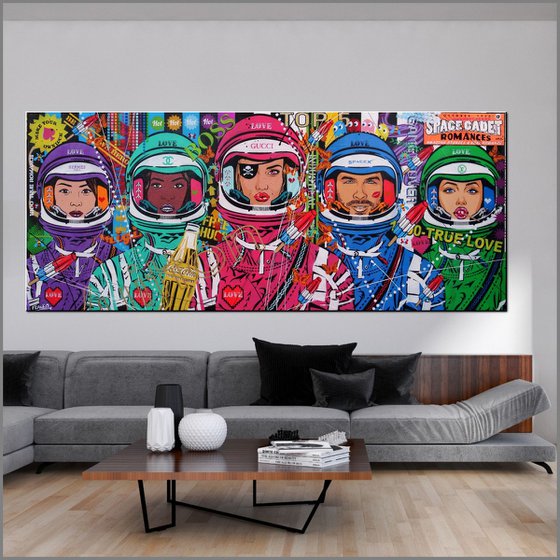The living room features an L-shaped gray suede sofa adorned with black throw pillows, some of which are positioned to allow the right side of the sofa to transform into a bed with an adjustable incline, similar to a hospital bed. The room's floor is a light-colored wood, complementing the space's bright and clean aesthetic. A large square coffee table with a black metal frame legs and a brown wood slab top sits in front of the sofa, decorated with a vase and a stack of magazines.

Dominating the white (though appearing slightly gray in the image) wall above the sofa is a striking, horizontally-aligned rectangular pop art painting. The artwork, which spans a very long poster frame, depicts five cartoon characters, each in different colored astronaut-style helmets and suits: from left to right, they are purple, green, pink (with an eye patch), blue, and dark green. The blue-suited character is the only male, while the others are women. The characters seem to represent different aspects of love, as indicated by the text; "true love" is printed across the green character on the far right, and the words "Space Cadet Romances" are prominently displayed at the top right of the painting. Some helmets feature brand names like Chanel and Gucci, adding a stylish touch to the whimsical illustration. This colorful and thematic artwork appears to be both a personal and aesthetic centerpiece in the room, reflecting the occupant's appreciation for comic-style pop art.